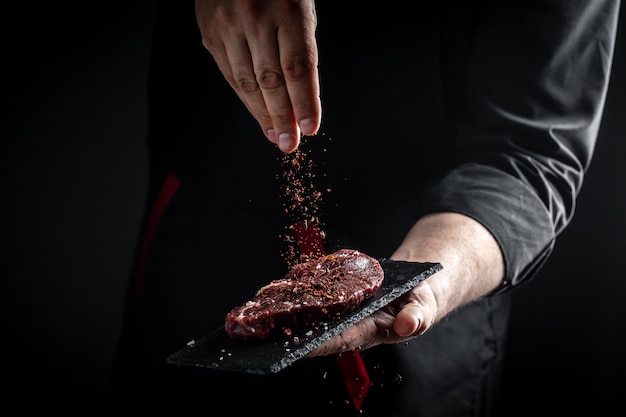The photograph captures a chef dressed in an all-black ensemble, including a long-sleeved black shirt with rolled-up sleeves and subtle reddish accents. He's positioned against a completely black background, enhancing the dark and dramatic theme of the image. The chef holds a small, black marble tray in his left hand, upon which rests a dark red, raw piece of meat, presumably a steak like a New York strip or prime rib. With his right hand, he is sprinkling a vibrant red, possibly Cajun, seasoning over the meat. As he does so, some of the seasoning flakes cascade onto the tray below. The meat appears to be boneless, and the light interplay casts shadows and highlights on the chef's sleeve and forearm, accentuating the image’s moody, high-contrast aesthetics.